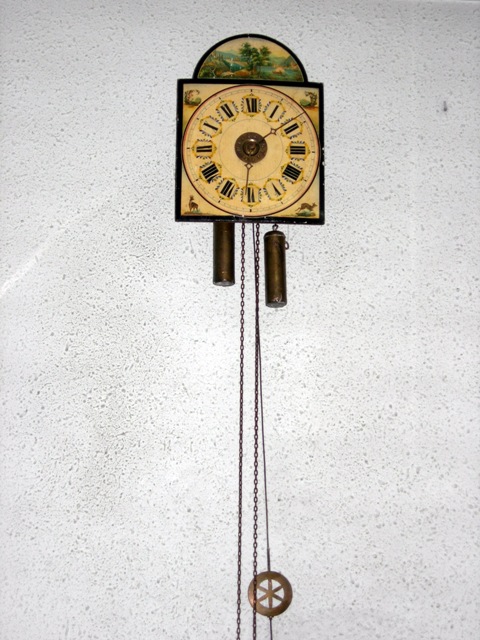The image features an old-timey square clock, prominently hanging on a light-colored wall with dark gray specks. The clock is situated close to the top center of the wall. At the top of the square clock is a semi-circle with an outdoor scene depicting trees, sky, and grass within a black border. Each corner of the square clock contains indistinct animal figures, likely deer, encompassed by a brown border.

The clock’s face displays Roman numerals, with black hands indicating a time of approximately 2:30. Below the clock are three long chains extending towards the bottom of the image. At the end of one chain is a circular ornament featuring a gold six-pointed star, while two dark gold-colored, cylindrical metal objects resembling bells or handles hang from the left and right sides of the chains. The overall design is accentuated by its intricate details and classic aesthetic.